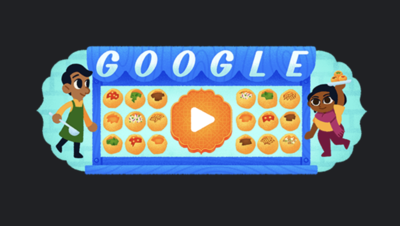This image is a captivating Google Doodle celebrating South Asian cuisine. Featuring a playfully animated scene, it showcases the Google logo atop a turquoise background adorned with intricate filigree detailing. The prominent blue signboard, with its large orange play button in the center, hints at an interactive game or animation.

On the left, a South Asian man in a yellow shirt, green apron, and black pants holds a ladle, ready to serve. Opposite him, a South Asian woman dressed in an orange shirt, burgundy pants, and a fuchsia scarf holds up a plate of delectable sweets. The eyes of both characters are notably large, adding to the illustration's cute and modern charm.

Surrounding the central play button is an arrangement of nine small pastries or bread bowls on each side, organized in a 3x3 grid pattern. These pastries are colorful and varied, some topped with red, green, or purple toppings, and others adorned with sprinkles and white sauce, resembling a delightful assortment of South Asian treats. The overall composition captures the festive and delicious spirit of South Asian culinary traditions.